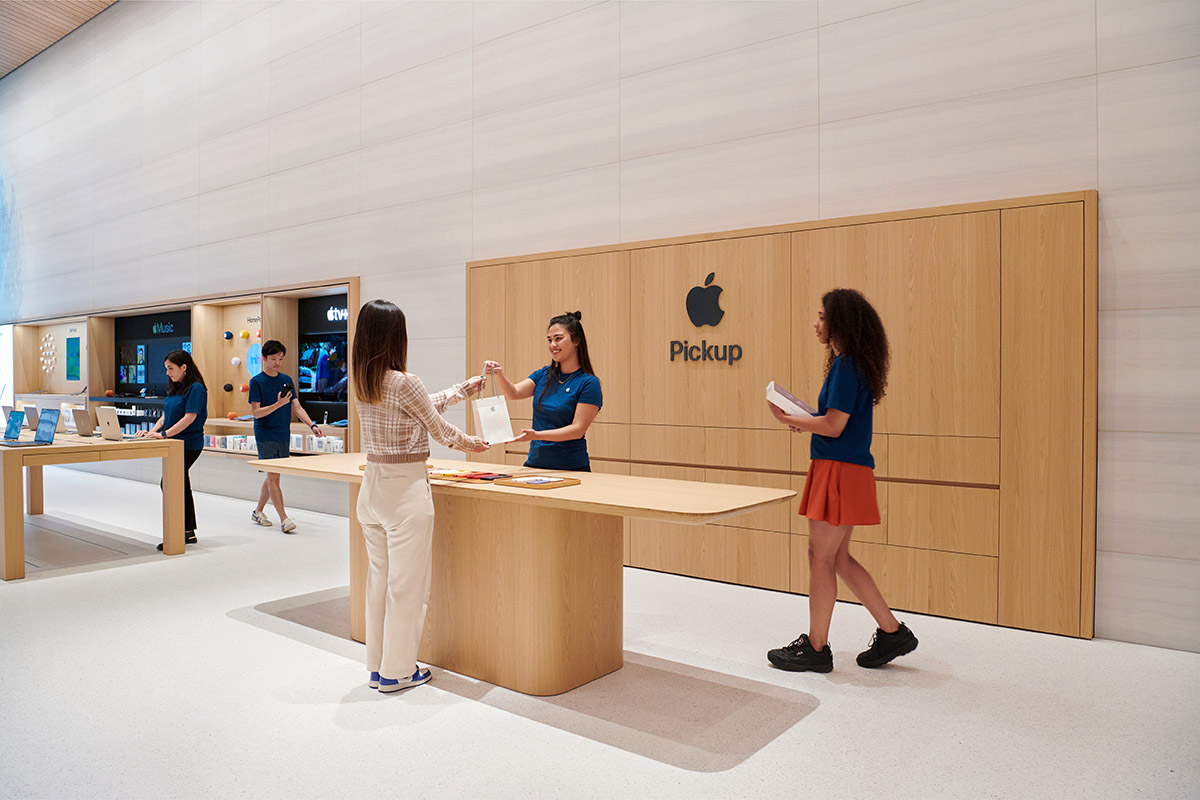An interior shot of a bustling Apple Store, showcasing a meticulously designed, modern space. The store features a pristine, white tiled floor and a tiled panel wall in a tan wood-like finish, creating a warm yet contemporary atmosphere. In the background, there are sleek oak-colored wooden displays, including one on the right with an "Apple Pickup" sign adorned with the iconic Apple logo, and another on the left spotlighting Apple Music and Apple TV.

Prominently, an oak table is situated in the foreground laden with laptops. Behind this table stands a young woman in a blue shirt, assisting customers. Central to the image is a distinctive desk-style table with a central base, extending wide on both sides, displaying various Apple products. A young woman with brown hair, also in a blue shirt, is handing a white gift-style bag to another woman dressed in a plaid top, white pants, and blue sneakers. Near them, a woman approaches holding a white box; she is attired in a blue shirt, orange skirt, and black shoes, adding to the lively, customer-oriented ambiance of the store.